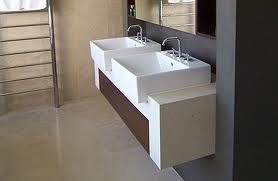The image depicts a compact public restroom with tan-colored walls and a grayish-tan tiled floor. On the left-hand side, there is a metallic structure resembling a step ladder with a white top. Adjacent to this, two white sinks are mounted on a white countertop, which has a brown base. Behind the sinks, a large mirror is set into the gray wall, reflecting the metallic structure and the surroundings. The gray wall extends to the right side, where it meets a black rectangular area that appears thicker at the bottom than at the top. The floor reflects both the metallic structure and the sinks. The sinks feature faucets with handles for hot and cold water, as well as a small drain opening at the top.